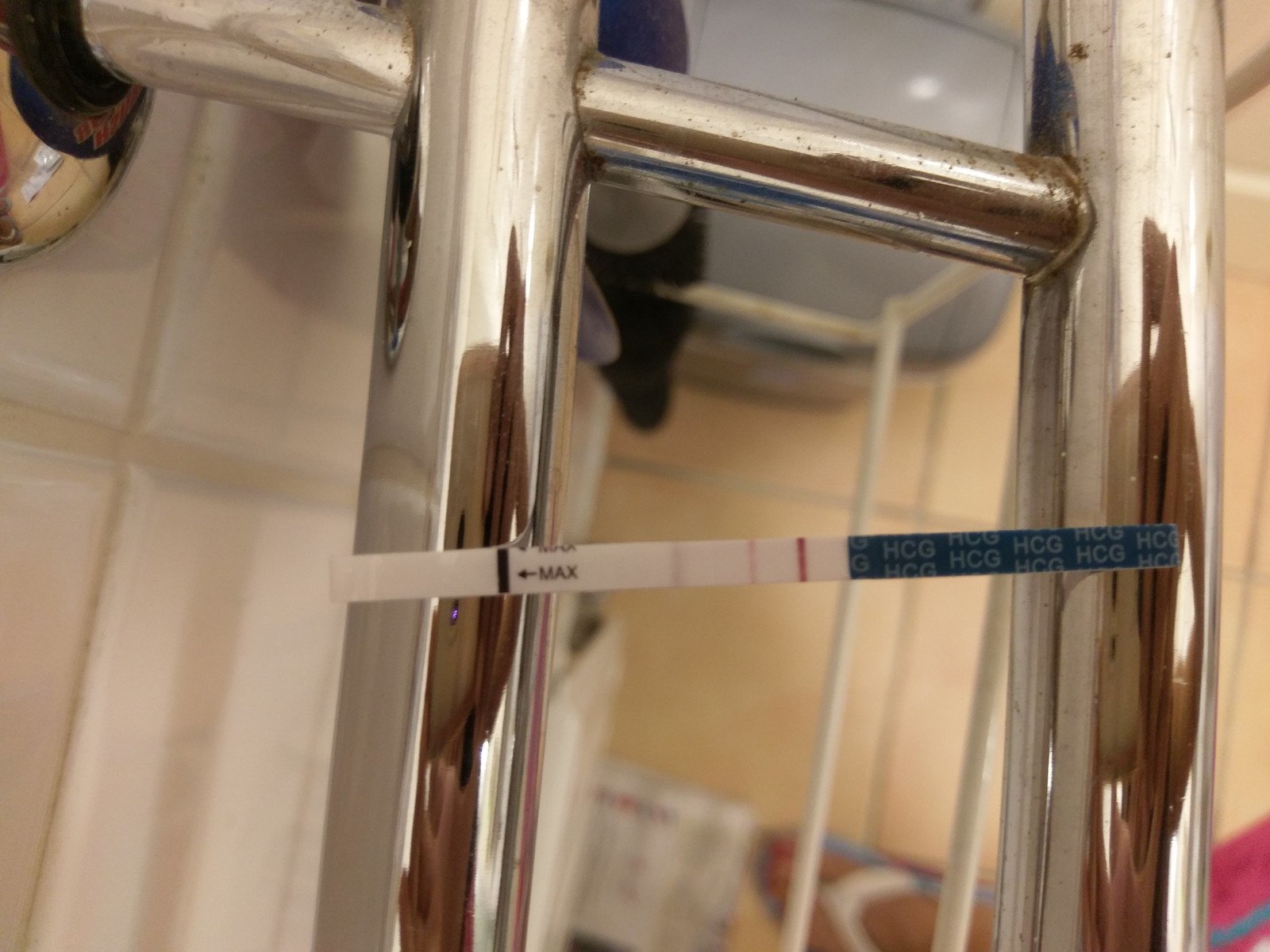The photograph, taken indoors, presents a bird's-eye view of a chrome towel rack mounted on a wall. The towel rack is affixed to a wall covered with white tiles and white grout, visible in the upper left corner of the image. These tiles extend into the background, occupying the left side of the frame before transitioning into a tan-tiled bathroom floor from the center frame towards the right edge.

In the background towards the top right corner, there is a glimpse of a blue trash can lid. The primary focus, however, remains on the chrome towel rack, which extends from its support in the upper left corner and is attached to two vertical chrome pipes. The left pipe is positioned just left of the center, while the right pipe is closer to the image's right edge. The towel rack and the pipes exhibit a slight rusting, and the photographer's reflection is noticeable in the chrome surface.

Dominating the lower half of the image is a thin plastic strip, approximately six inches long and half an inch wide, draped over both bars of the towel rack. The strip is predominantly white on one side and blue on the other, with the word "max" printed alongside an arrow pointing to the left, and a blue vertical stripe to the left of the text.